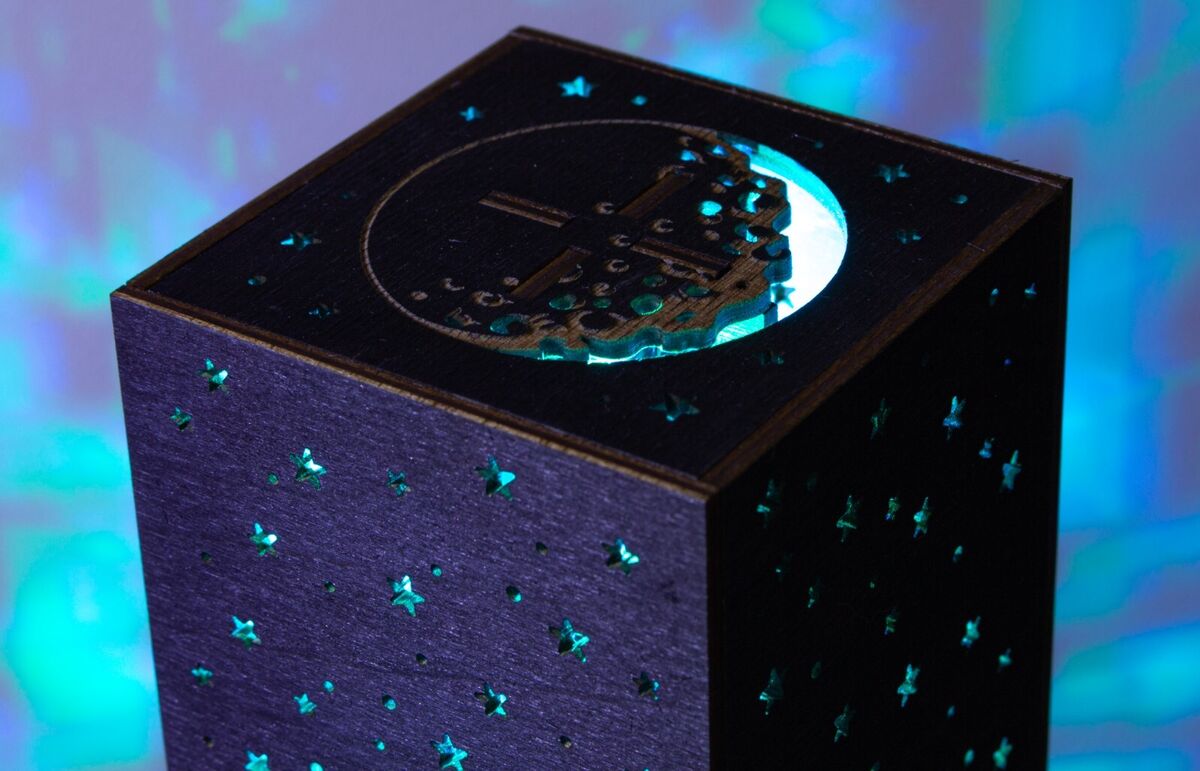The image features a cube-shaped box positioned at an angle, allowing a view of its top surface and two of its sides. Against a glowing purple and blue background, the box appears almost black but is illuminated from within by a bluish light that seeps through various cutouts. The top surface showcases a circular cutout resembling a half-moon shape, revealing a glowing internal light. Additional star-shaped cutouts of varying sizes perforate the top edge and all visible sides of the box, enhancing its luminescence. The emitted light casts an iridescent blue and green glow on the surrounding walls, creating a striking ambiance.